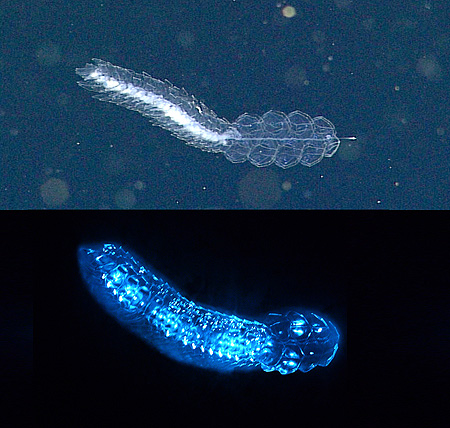This image consists of two parts, each depicting the same microorganism from different perspectives. The top drawing features a dark blue background with goldish-yellow circles, some vibrant while others are faded. The microorganism, against this backdrop, has a clear membrane filled with various circles concentrated on the right-hand side, tapering into a spiky tail with a central white line, resembling a skeletal or x-ray view. The bottom drawing showcases the same organism in a more photorealistic manner; set against an almost black background, it emits a bright blue bioluminescence, especially pronounced at the center. The organism is worm-like with a bullet-shaped head and a tapering tail. The translucent membrane and internal structures are illuminated, creating a striking contrast with the dark environment, making it look like it was captured underwater.